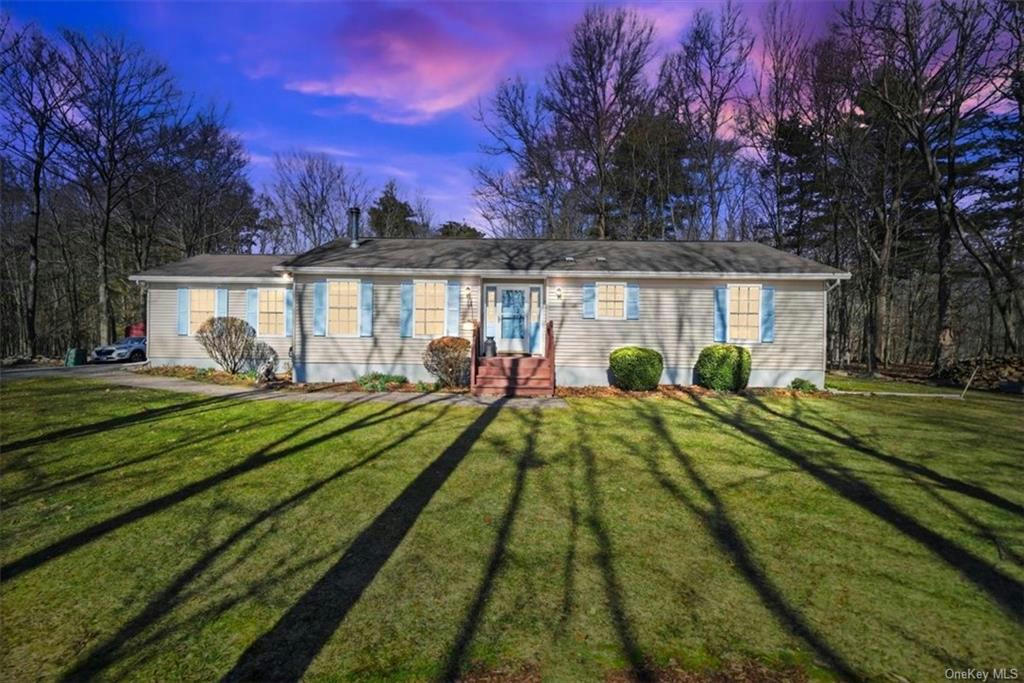The image showcases a detailed 3D color illustration of a single-story house set against a captivating, late-evening sky. The sky is a striking blend of vibrant blue with tinges of purple, reflecting off the clouds, adding a surreal touch. Positioned centrally, the house features a gray shingle roof with blue shutters adorning its windows. The structure is clad in white-gray horizontal siding, with a blue front door accessed by brown wooden steps. 

On either side of the door are six windows in total: four identical ones to the left and two on the right, including one shorter and one taller window. A side-entry garage is visible on the left, highlighted by two additional blue-shuttered windows and a few parked cars. Bushes line the foundation, with wilted ones on the left and lush green ones on the right.

The surrounding wooded area casts elongated, somewhat eerie shadows of unseen trees across the foreground’s grassy lawn, hinting at a Halloween-like atmosphere. Lastly, the distant colorful clouds framed by dark green trees bracket the house, completing the serene yet intriguing scene.